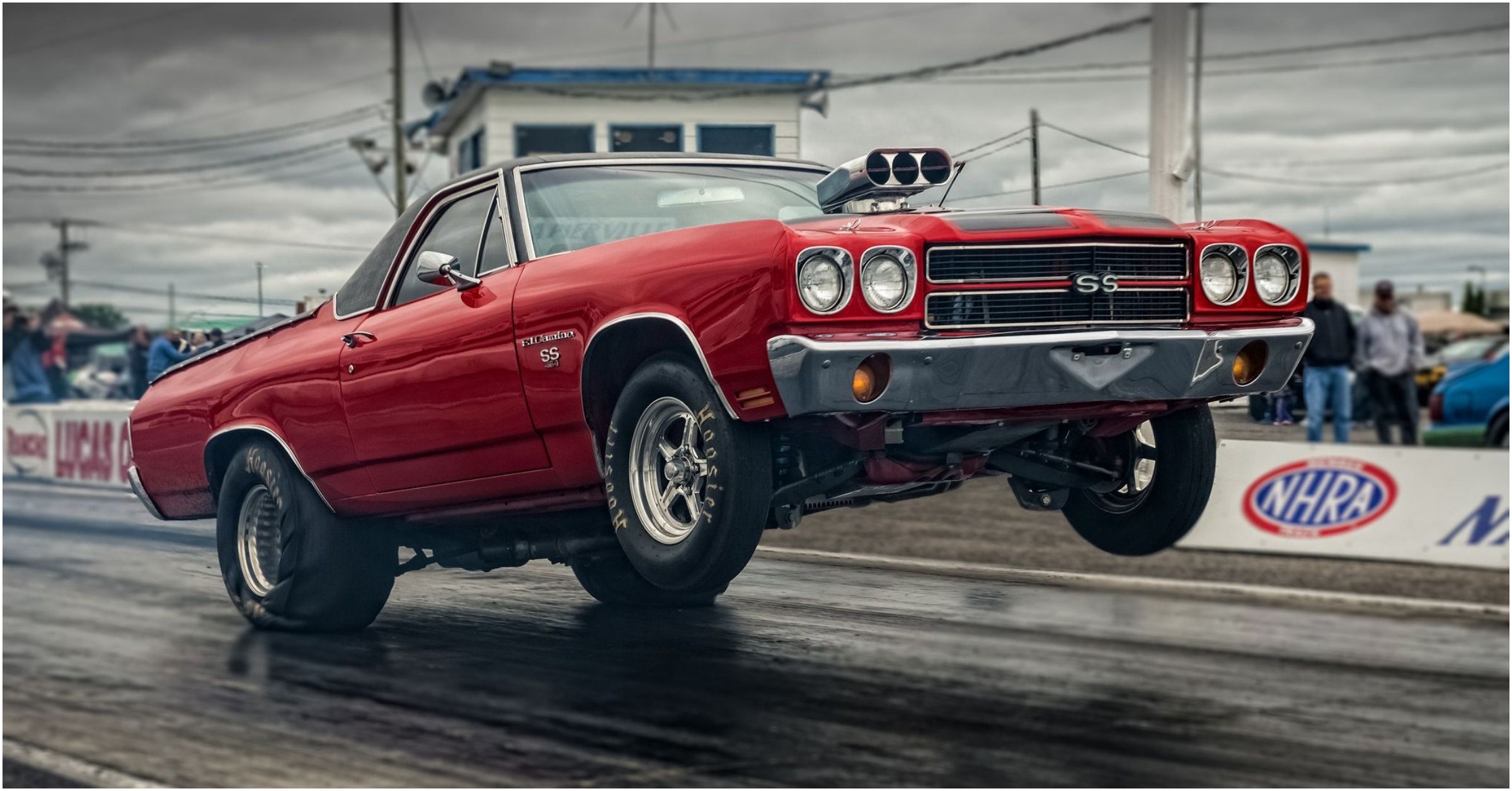This photograph captures a vivid scene at a speedway, showcasing a bright red, retro muscle car, possibly from 30-40 years ago, with a striking SS emblem on its front grille. The car is turbocharged, as evidenced by the protruding engine modification on its hood. The image captures the car in mid-action, with its front wheels lifted off the ground, performing a dramatic wheelie on its shiny chrome-rimmed back wheels. The car is adorned with four black wheels and a black soft top, hinting at its convertible nature. 

Gray, stormy skies loom overhead, suggesting it might have just rained. The backdrop features the NHRA (National Hot Rod Association) symbols, reinforcing the racing atmosphere. People are scattered around the speedway; to the far right, some are staring off into the distance, while others on the left appear to be conversing or working, though their faces are out of focus. A speedway rooftop and a blurred tower are visible behind the car, further situating this thrilling moment firmly within the racetrack environment.